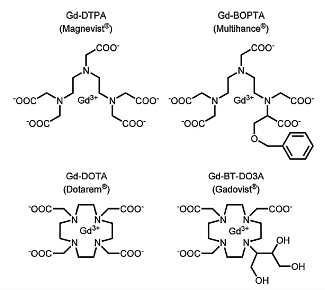The image is a detailed scientific diagram featuring four distinct molecular structures, each indicative of various gadolinium-based contrast agents used in medical imaging. Positioned on a white background, the diagrams are arranged as follows: at the upper left is GD DTPA labeled as Magnevist; to the upper right is GD BOPTA labeled as Multihance; at the bottom left is GD DOTA labeled as Doterem; and at the bottom right is GD BT DO3A also labeled as Magnevist. Each molecule showcases a complex structure with nitrogen (N) at the center connected to various carbon (C) and oxygen (O) compounds, resembling geometric or honeycomb-like patterns. Text annotations identify the molecular structures and their respective labels. Notably, the diagrams include COO groups and variations in their structural connections. The GD BOPTA (Multihance) and GD BT DO3A (Magnevist) show additional elements and unique structural differences compared to the others.